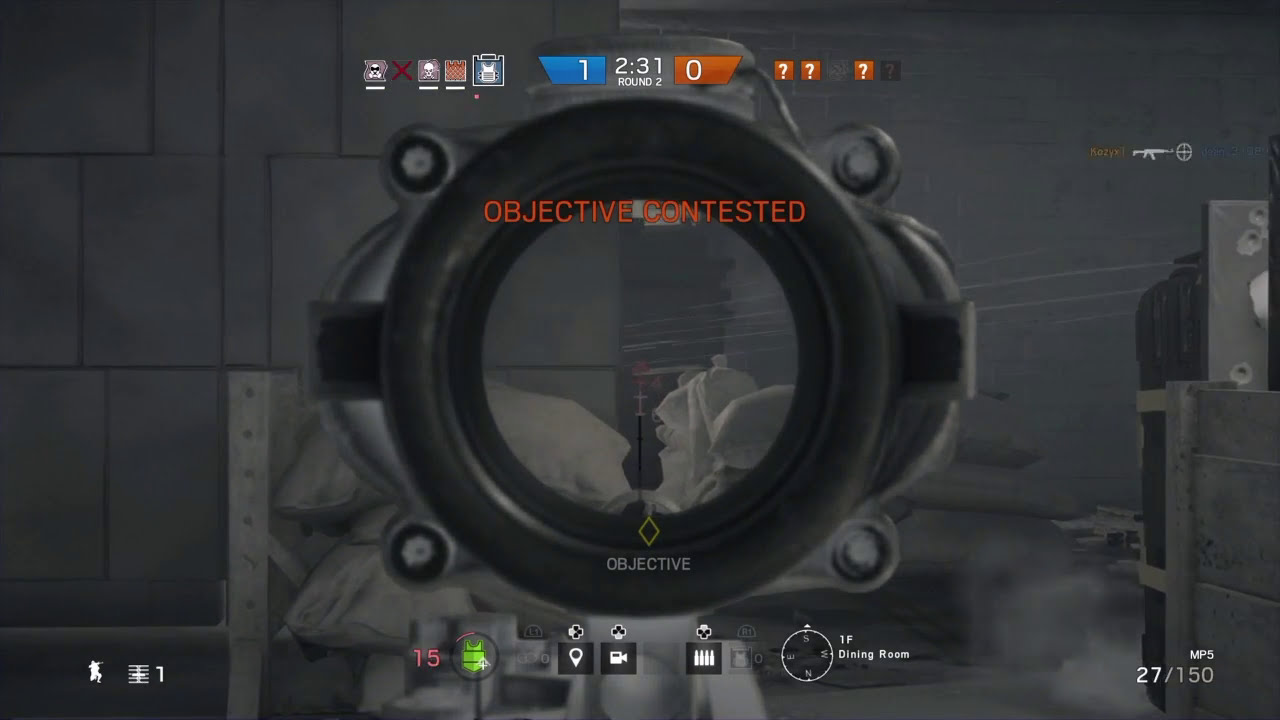The image is a detailed screenshot from a first-person shooter video game, portraying a dark, gray-toned scene. Dominating the foreground is a circular, black-and-gray scope, possibly from a sniper rifle, with small bolts on each side of it and a yellow crosshair in the center. The scope magnifies a section of the background, revealing scrunched-up white bed sheets and a steel bed frame or cot, suggesting a prison cell or similarly stark environment. Above the scope, orange text reads "Objective Contested," which is reiterated in some descriptions as yellow. Below the crosshair, white text indicates "Objective."

At the top of the screen, there's a status banner for the game round, displaying the score with the blue team leading 1-0 against the orange team, and a timer showing 2 minutes and 31 seconds remaining in Round 2. To the right of the score and timer, orange question mark icons are visible. The bottom right corner features an MP5 gun icon, along with ammunition count displaying 27 out of 150 rounds. Additional icons, including a compass showing "N, S, E, W" points, along with the text "1P" or "1F Dining Room," are visible below the scope, providing further navigational details to the player.